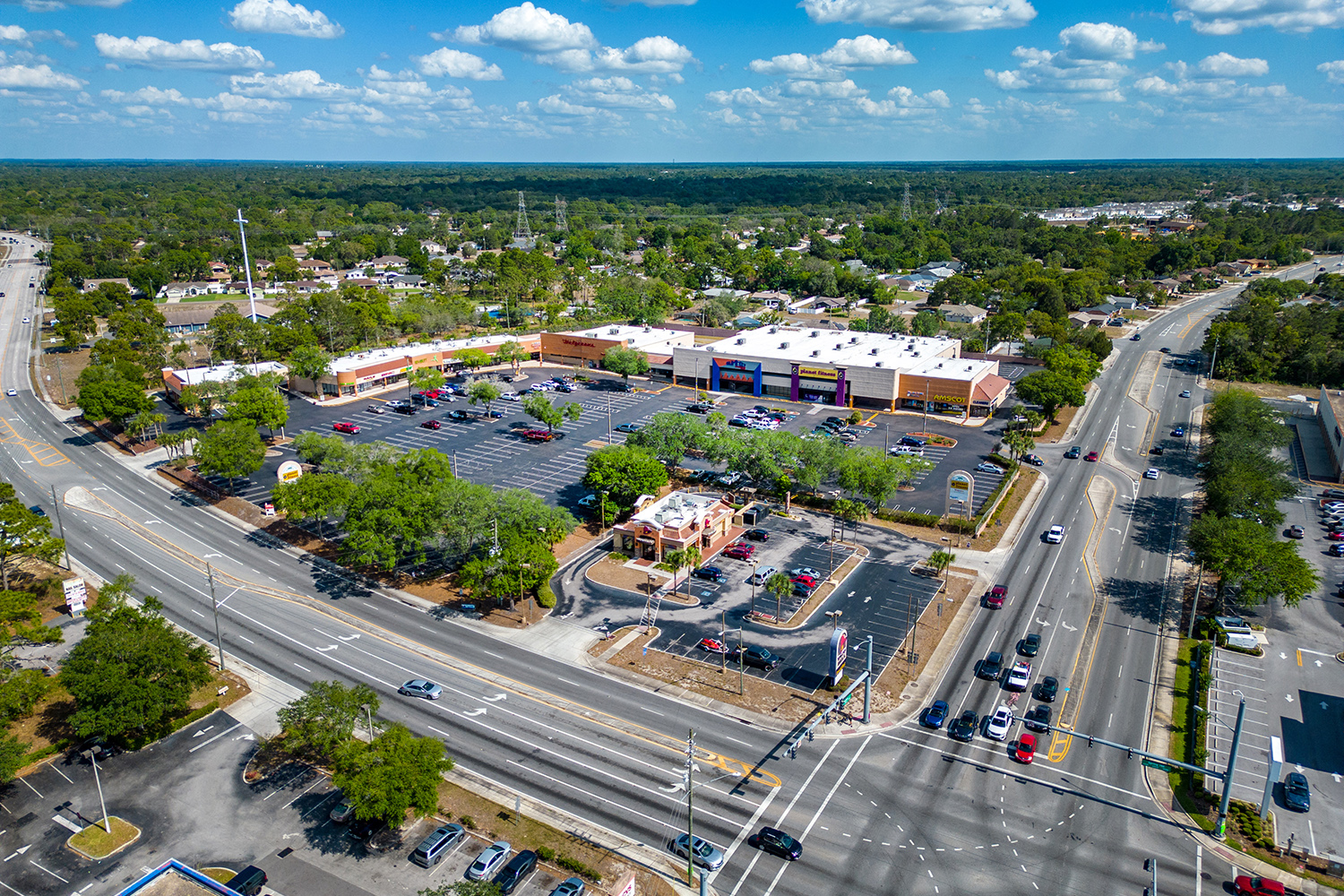The photo is an aerial daytime view of a bustling area with a strip mall complex at its center. The foreground is dominated by a large black parking lot with clearly marked white parking spaces. This parking lot sits in front of a strip mall housing various stores, including recognizable names like Walgreens, Planet Fitness, and Amscot, although many store signs are too distant to read clearly. On the far right and bottom left of the image, additional parking lots are visible, filled with numerous cars and framed by traffic lights. 

The left side of the image features a roadway that extends almost to the top, while another road appears on the right side, also stretching towards the upper section of the frame. Trees are strategically placed in front of the parking lot and along the roads, adding greenery to the urban landscape. Beyond the strip mall, the land transitions into a vast expanse of green trees. Around 80% up the image, the horizon line marks the edge of the tree-filled land below a clear, light blue sky dotted with fluffy white clouds. In the bottom right, a significant intersection is visible, connecting the area’s roadways. The overall view captures the essence of a busy, suburban shopping area surrounded by natural scenery under a beautiful, partly cloudy sky.